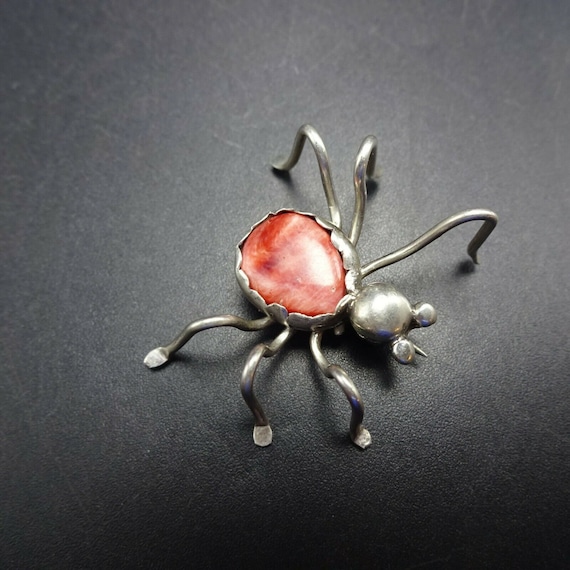This photograph features a detailed and artistic piece of jewelry, likely a brooch, shaped to resemble a beetle or spider. The central element of the piece is a teardrop-shaped red stone with a marbled appearance, showcasing a blend of red and white swirls. The stone has a polished finish and is firmly secured by fine silver flaps that curve around it. The jewelry piece is meticulously crafted, with six silver wires extending from the stone to form the bug's legs. The beetle's head is round and has two small, rounded protrusions resembling ears. The overall design appears to be made from silver, and the image shows a slight hint of a pin between the "ears," suggesting that this is indeed a brooch intended to be worn on a lapel. The backdrop is a stark black, making the metallic and stone elements stand out vividly.